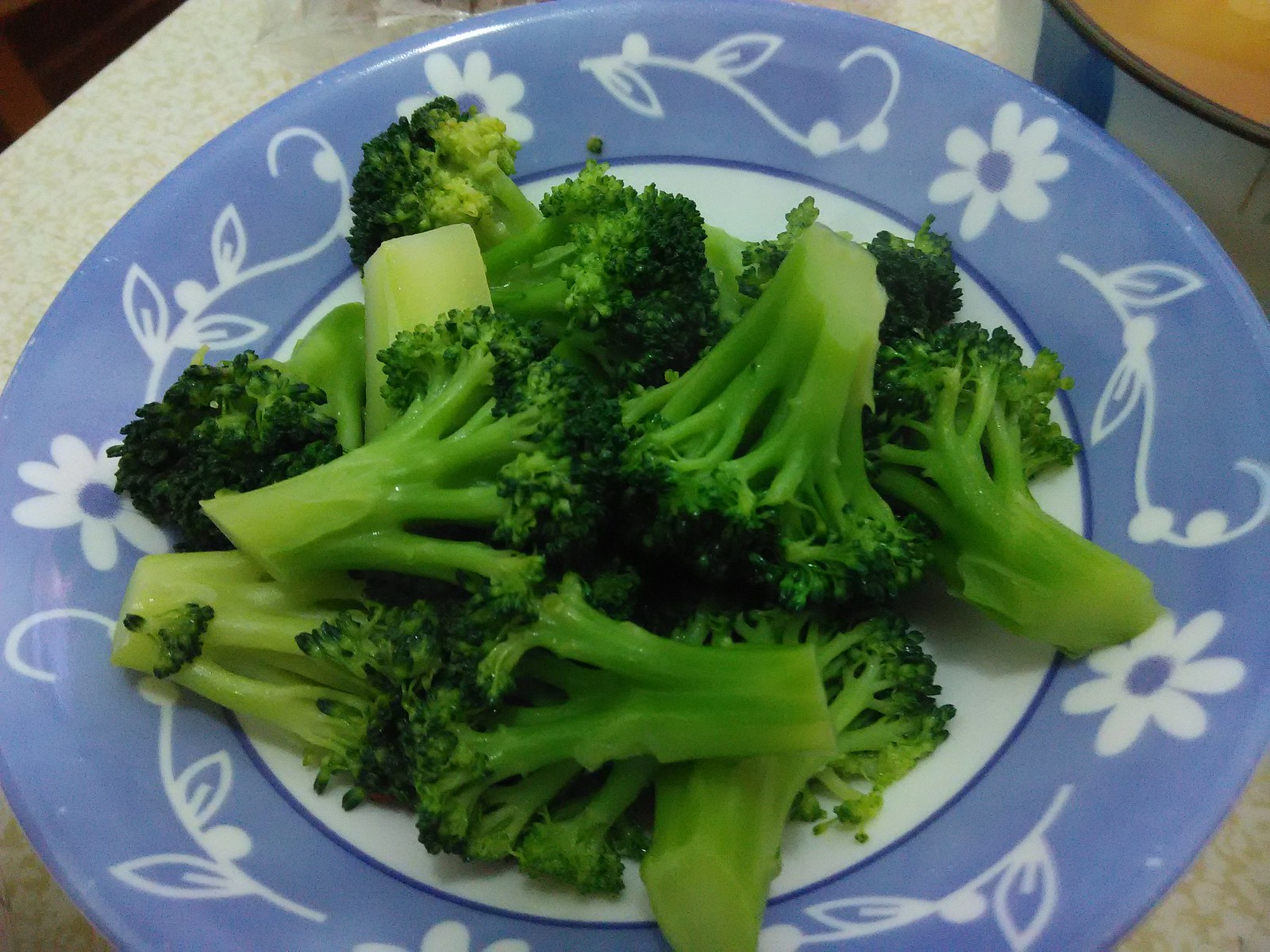A close-up image captures a white table supporting a blue and white ceramic plate heaped with freshly washed and chopped, vibrant green broccoli. The plate's design features a white center bordered by a light blue rim, with intricate white floral patterns set against the blue background. The juxtaposition of the strikingly green broccoli against the detailed, colorful plate makes for a visually compelling composition. The table behind the plate is barely visible, emphasizing the dominant presence of the plate and its contents in the photograph.